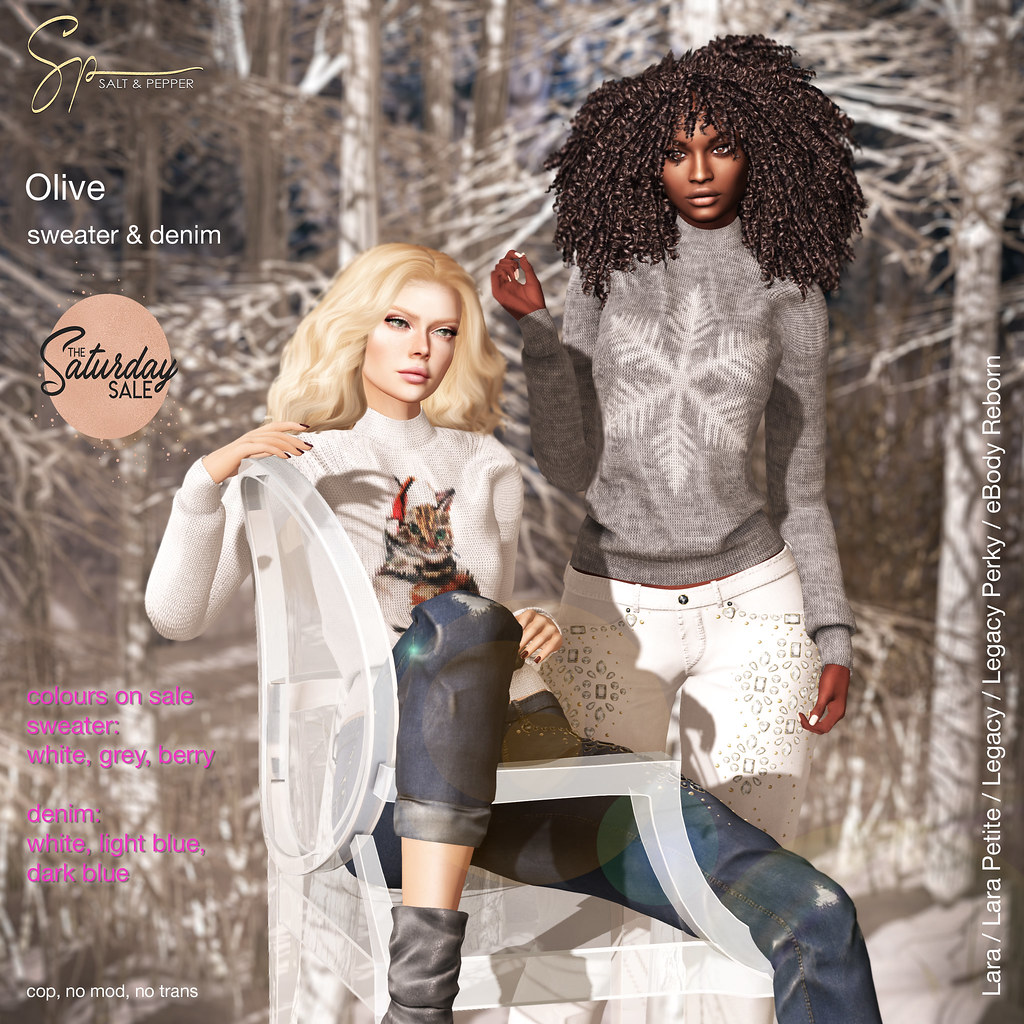The image is a detailed computer-generated advertisement for a company, possibly named "Salt-N-Pepper," promoting a "Saturday Sale" on denim and sweaters. The scene is set outdoors against a background of a forest with trees, lending a wintery atmosphere to the display. The advertisement features two mannequins with distinct appearances and attire. On the right side stands an African-American mannequin with beautiful long curly hair, dressed in a gray sweater adorned with a snowflake design, and white jeans that appear to have rhinestones. To the left, sitting in a chair with her legs draped over the armrest, is a Caucasian mannequin with very blonde hair. She is dressed in jeans and a festive white sweater featuring a cat wearing a Santa Claus hat. The mannequins have blank expressions, emphasizing the clothing rather than the characters. Text on the left side of the image mentions "Salt-N-Pepper," "Olive, Sweater, and Denim," and highlights the "Saturday Sale," indicating the colors and types of denim available for the promotion.